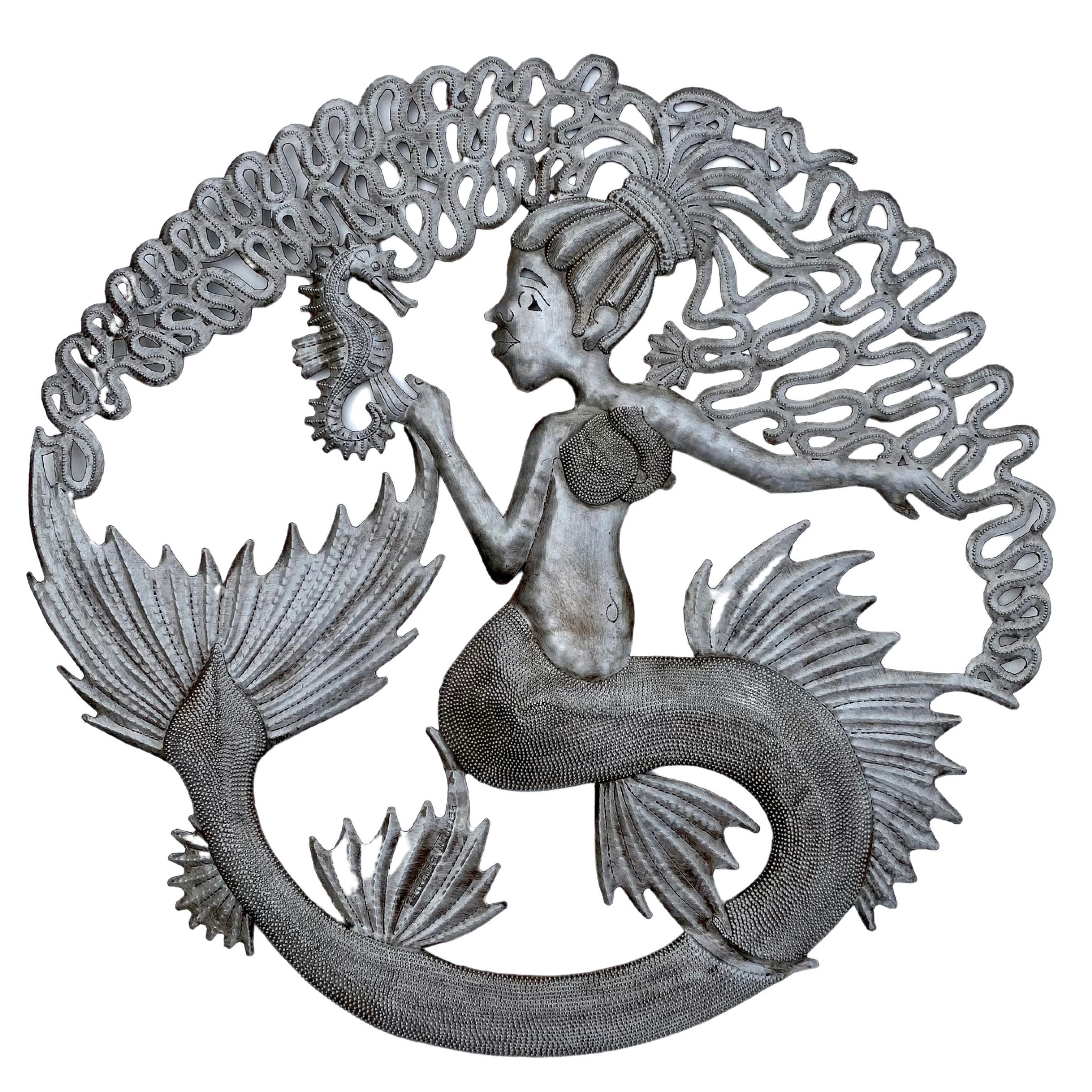This detailed metal artwork showcases a mermaid centered in a circular design, made entirely of silver-toned metal. The mermaid's long, dread-like hair encircles the top of the piece, emerging from a ponytail bound with a band on the top of her head. Her hair streams outward in intricate, squiggly strands, creating a continuous flow into her giant fish tail, which spirals around the bottom of the design and completes the circle on both sides. 

She is depicted looking to her left, her face partially visible, focusing intently on a detailed seahorse held in her right hand. The seahorse's tail rests in her open palm, and its head touches her flowing hair. The mermaid's left arm extends outward, with her hand open and facing downward. Her body is adorned with a darker metal bikini top, leaving her midriff exposed before transitioning into her ornate, scaled tail that winds gracefully across the whole bottom section of the artwork. The composition balances the mermaid's intricate details, the texture of her scales, and the dynamic flow of her hair and tail, producing a captivating and harmonious piece of metal art.